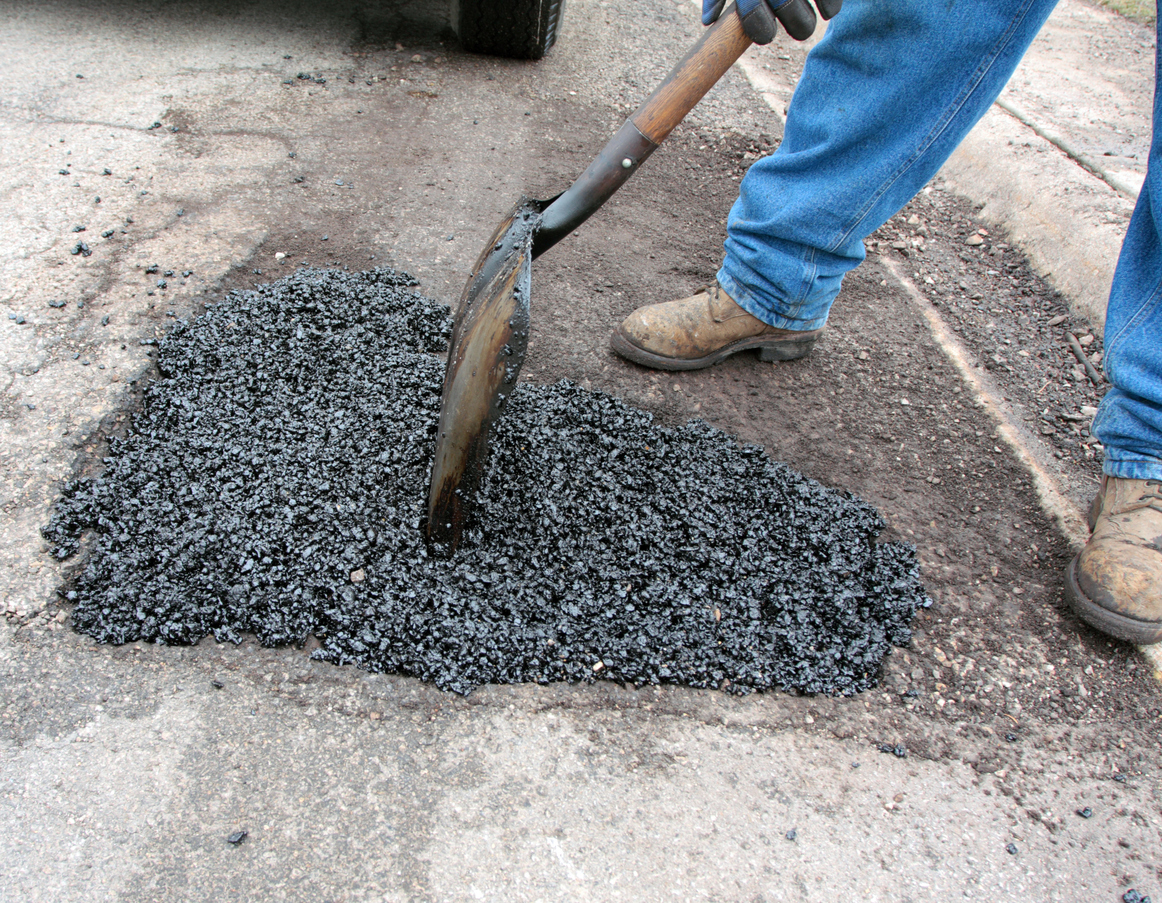This photograph captures a man in mid-action, working to repair a street next to the curb. Dressed in well-worn but sturdy work boots, denim jeans, and thick gloves, the man appears to be an experienced laborer, possibly a worker from the Department of Water and Power. He is using a well-used square-nose shovel with a dark wooden handle, diligently packing down a fresh layer of dark black, shiny asphalt to fill a pothole. The asphalt looks hot, suggesting it has just been poured. The scene is set during the daytime under an overcast sky, as there are no visible shadows. The street itself is in a state of disrepair, with visible cracks and scattered gravel, indicating it has been neglected for some time. Partially cut off in the frame, a tire—likely from a cart or truck—hints at nearby equipment or a vehicle parked out of view, contributing to the ongoing repair work.